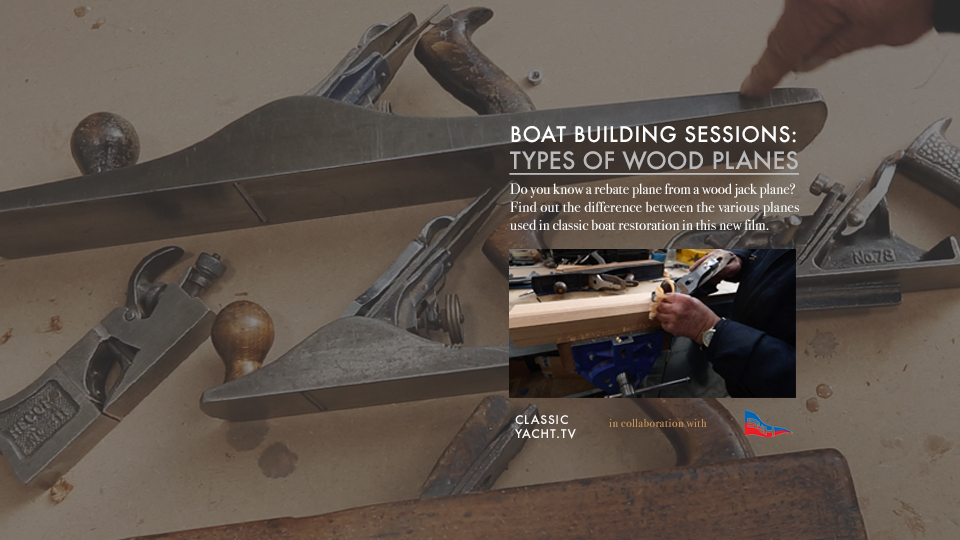The image is a detailed graphic advertisement for a film on classic boat restoration techniques. At the center, the text in white reads: "Boat building sessions. Types of wood planes. Do you know a rebate plane from a woodjack plane? Find out the difference between the various planes used in classic boat restoration in this new film." The background features various wooden and metal tools, prominently showcasing wood carving or building tools. Below the text, there is a rectangular photograph displaying a man's hand expertly shaving a piece of wood with a plane. To the bottom left of the image, the text "classicyacht.tv" is visible, indicating collaboration with another organization, represented by a blue and red flag on the right side.